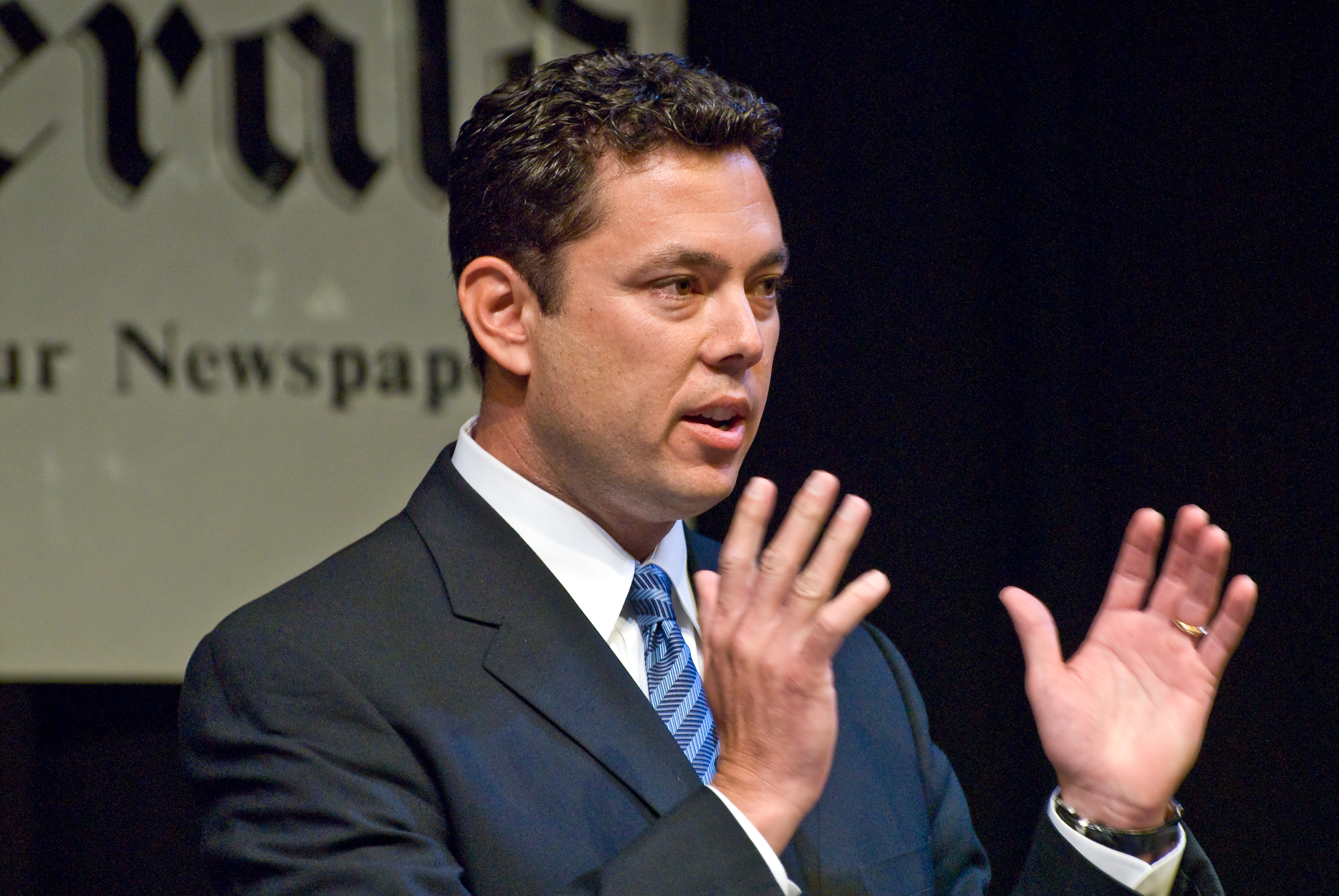In the image, there is a man positioned directly in the center, appearing to speak at a public assembly or presentation in a dimly lit indoor setting. The background is predominantly black and blurred, with a hint of a poster or newspaper visible in the upper left corner. The man, who has dark, styled hair, is wearing a navy suit, a white shirt, and a tie with alternating light blue and dark blue zigzagging stripes. He appears to be gesturing with his hands raised, showcasing a wedding ring on his finger and a watch with a black band on his wrist. The colors in the image include various shades of black, gray, off-white, white, and blue. There is no discernible text in the background aside from the partial poster which might say "Harold" and mention something about a newspaper.